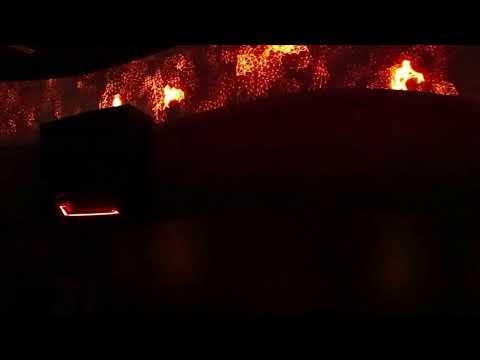The blurred nighttime photograph presents a surreal, almost abstract scene dominated by dark tones and sporadic patches of red light. The left side features a prominent black box-like structure, highlighted by a stark red LED strip at its bottom, suggesting the entrance to a chute. Both the bottom section of the image and the top are framed by black rectangular borders, contributing to the overall mysterious ambiance. Within the lower part of the image, two indistinct, pixelated faces emerge from the darkness. Contrary to the overall obscurity, the top section mesmerizes with vivid, fiery imagery - bright orange and yellow flames, interspersed with streaks of red and black, stretching upwards in various shapes and sizes. This part of the image lacks any indication of actual burning, suggesting it might be a decorative element. To the left, a small but sharp red light punctuates the image, while the top right corner intriguingly hints at a humanoid figure formed by white light against a red, textured background. This intricate mix of dark and light elements, coupled with unusual textures and shapes, evokes an enigmatic and almost otherworldly scene.